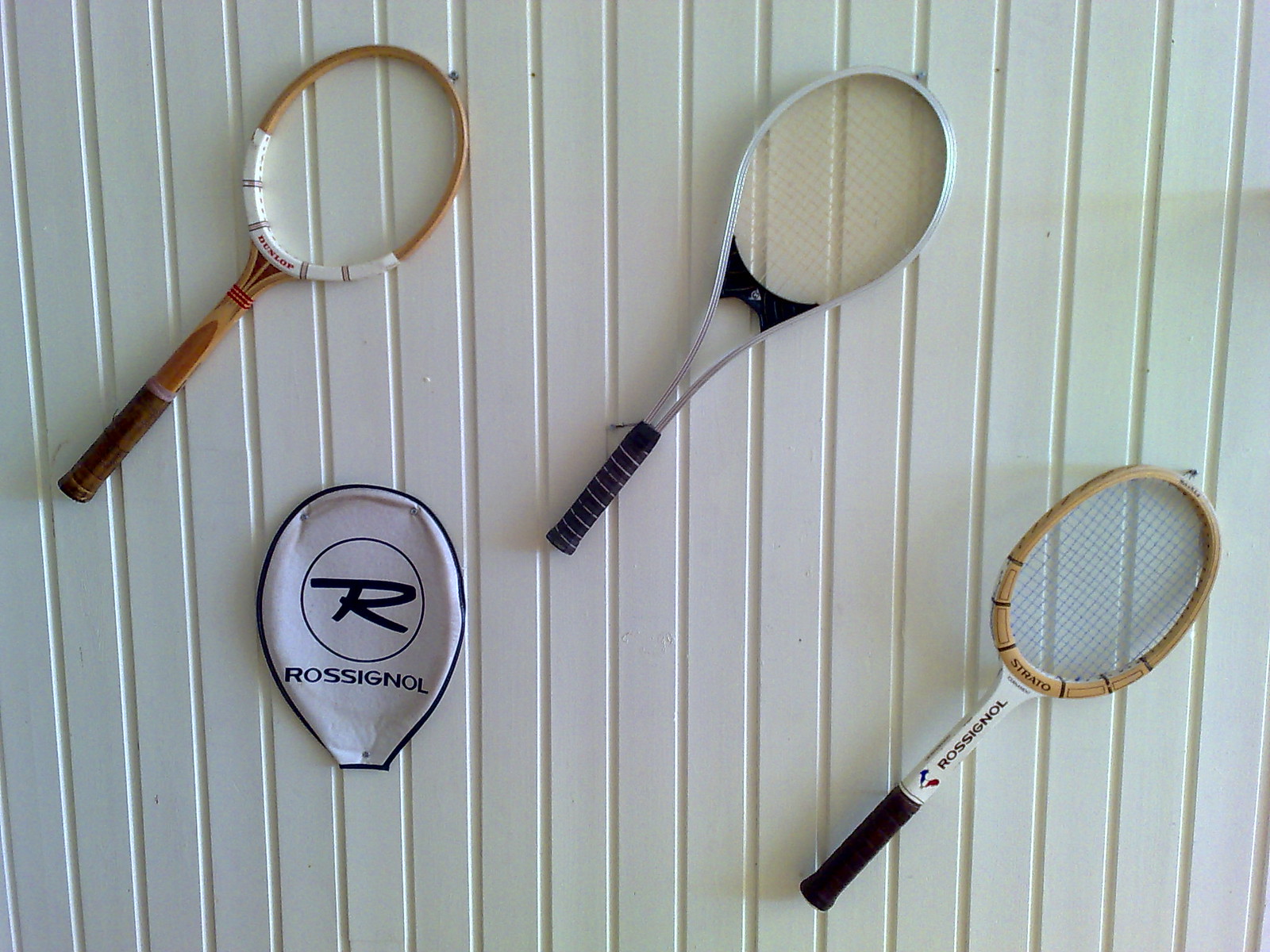This vibrant color photograph captures a trio of vintage tennis rackets mounted diagonally on a white, paneled wall with vertical ridges. The bright sunlight suggests it may have been taken indoors near a window. The rackets are arranged with their handles pointing to the lower left and their heads to the upper right. The upper left racket is an old wooden model featuring a frame with red "Dunlop" lettering where the handle meets the neck. The center racket, slightly elevated and to the right, is metal with a black grip. The lower right racket is another wooden model with a black grip, displaying the word "STRATO" at the neck. Underneath the top two rackets is a white racket cover with blue trim, prominently branded with a circular "R" logo and the name "Rossignol" beneath it.